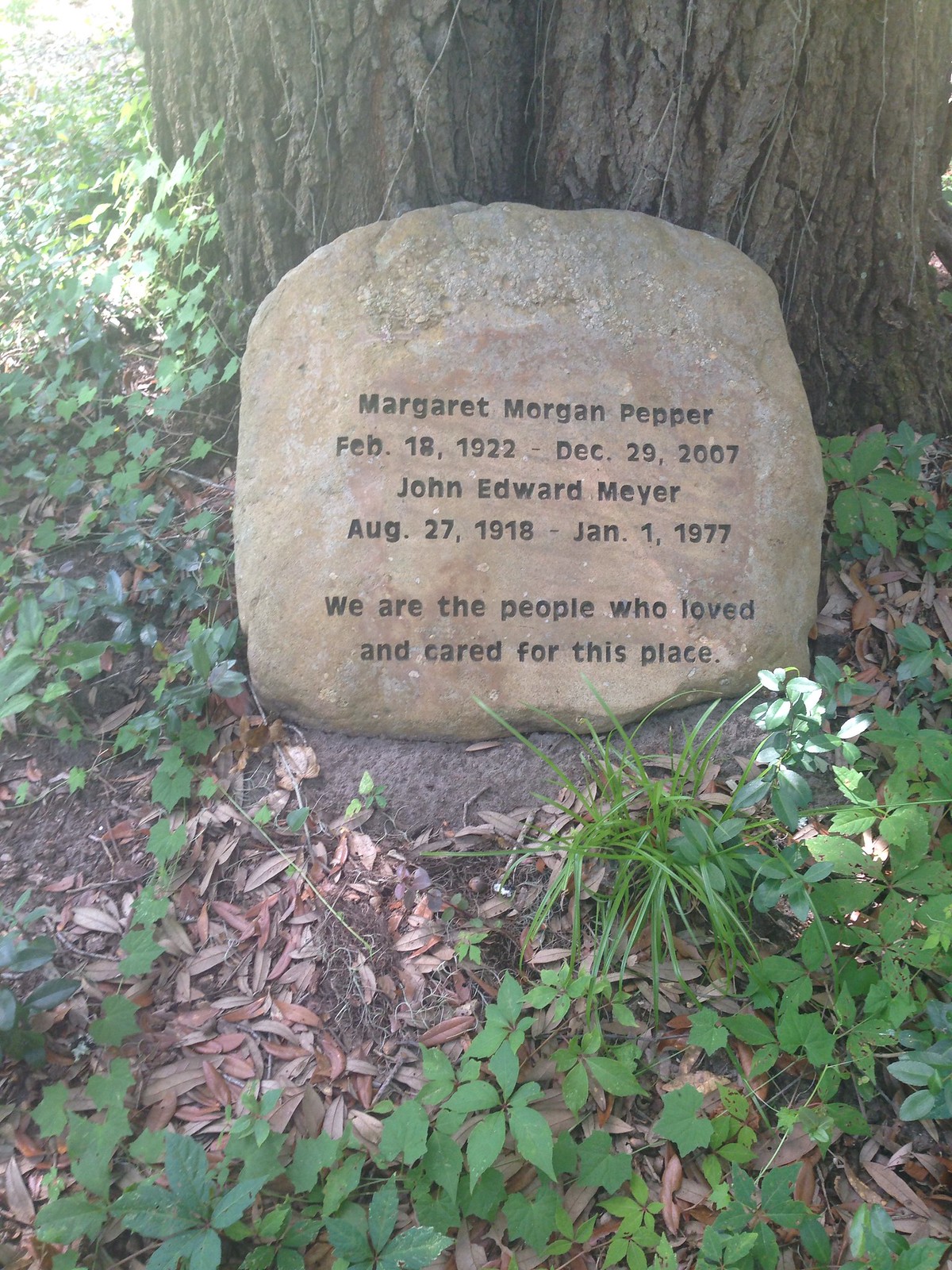The image depicts an outdoor scene with a large tree and abundant green foliage. Laying against the base of the tree is a tan-colored boulder with faint gold streaks, which serves as a tombstone. Carved into the stone in black text are the names and dates: "Margaret Morgan Pepper, February 18, 1922 - December 29, 2007," and "John Edward Meyer, August 27, 1918 - January 1, 1977." Below the dates, an inscription reads, "We are the people who loved and cared for this place." The stone is surrounded by leaves, ivy, and wild blackberry plants, giving the impression that the scene is set in a serene forest or park, with the tombstone being a heartfelt memorial to those who cherished the area.